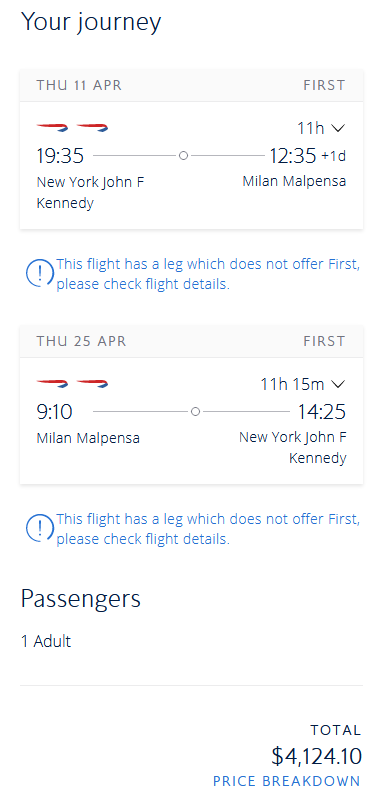This screenshot captures a flight booking application interface. The layout suggests it is an active booking within the app, primarily displayed on a minimalist white background. 

At the top, the title "Your Journey" is prominently shown. The screen is divided into sections detailing departure and return flights, each section underscored with a light gray outline and featuring a banner with the respective dates.

The first flight, departing on Thursday, April 11th, is scheduled to leave New York at 19:35 and arrive in Milan at 12:35 the following day, making for a total travel time of 11 hours. 

The return flight is set for April 25th, departing Milan at 09:10 and landing back in New York at 14:25.

Each flight detail includes a blue icon with an exclamation point, accompanied by a note in blue text that reads: "This flight has a leg which does not offer first class. Please check flight details."

Beneath the flight information, the passenger count is listed as "1 adult." On the right side, the total cost for the round-trip ticket is displayed: $4,124.10. A blue clickable link labeled "Price Breakdown" is available for users to view the detailed fee structure contributing to the total fare.

The specific booking service or app name is not mentioned, focusing instead on the final price breakdown for the round-trip itinerary.